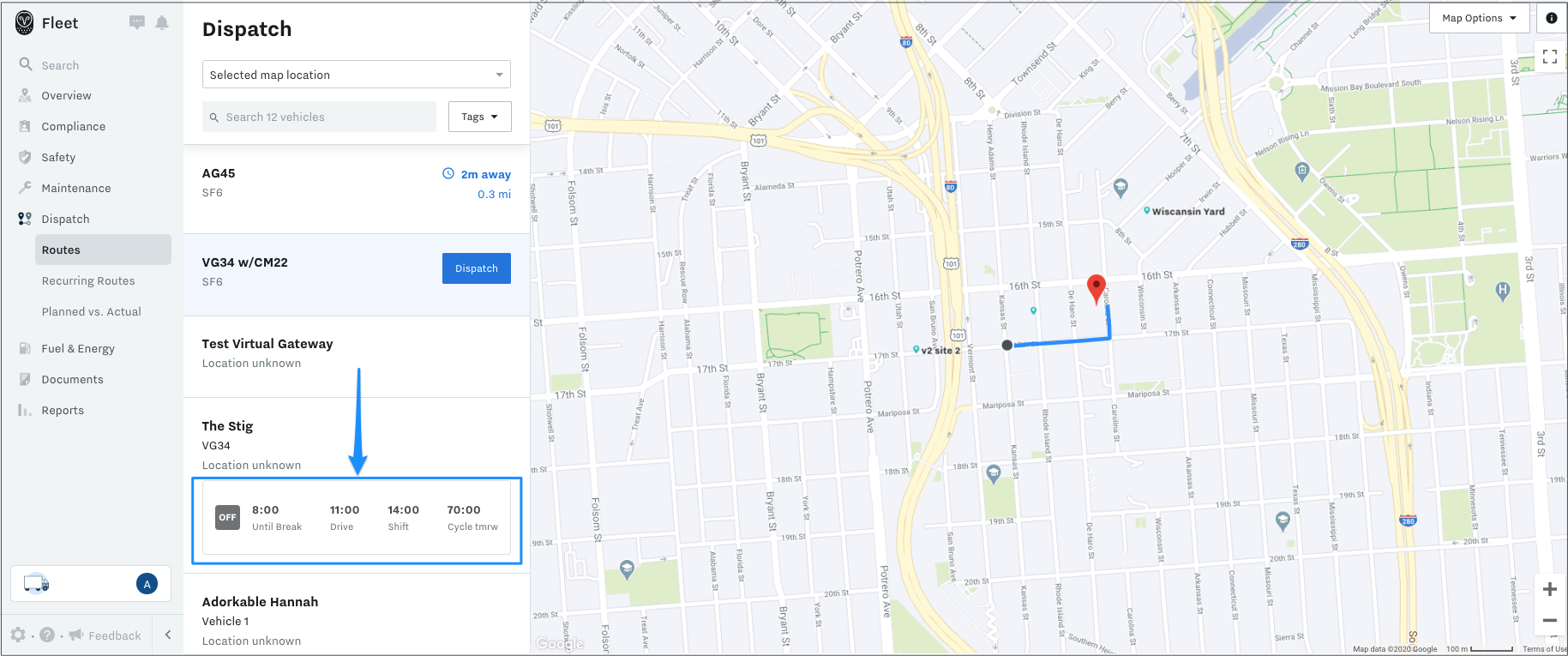In this image, the right side is dominated by a Google map interface featuring a prominent red location icon, a blue route line extending from the icon, and ending at a small black circle. The map is detailed with geographic and navigation elements. On the left side of the image, an organizational menu labeled "Fleet" sits at the very top left. This menu is vertically aligned and comprises several categories including Search, Overview, Enterprise, Safety, Maintenance, Logitech, Fuel and Energy, Documents, and Reports. At the bottom left of this menu is a white rectangle containing a blue circle with the letter 'A' and an icon of a truck driving to the right. Additionally, there are functional icons for settings and help just below the search bar. At the very top right corner, the word "Dispatch" is displayed prominently. Below this, two search bars are positioned; the top one with the placeholder text "Select Map Location" and the bottom one with the placeholder text "Search Vehicles," accompanied by the word "Tags" to the right.